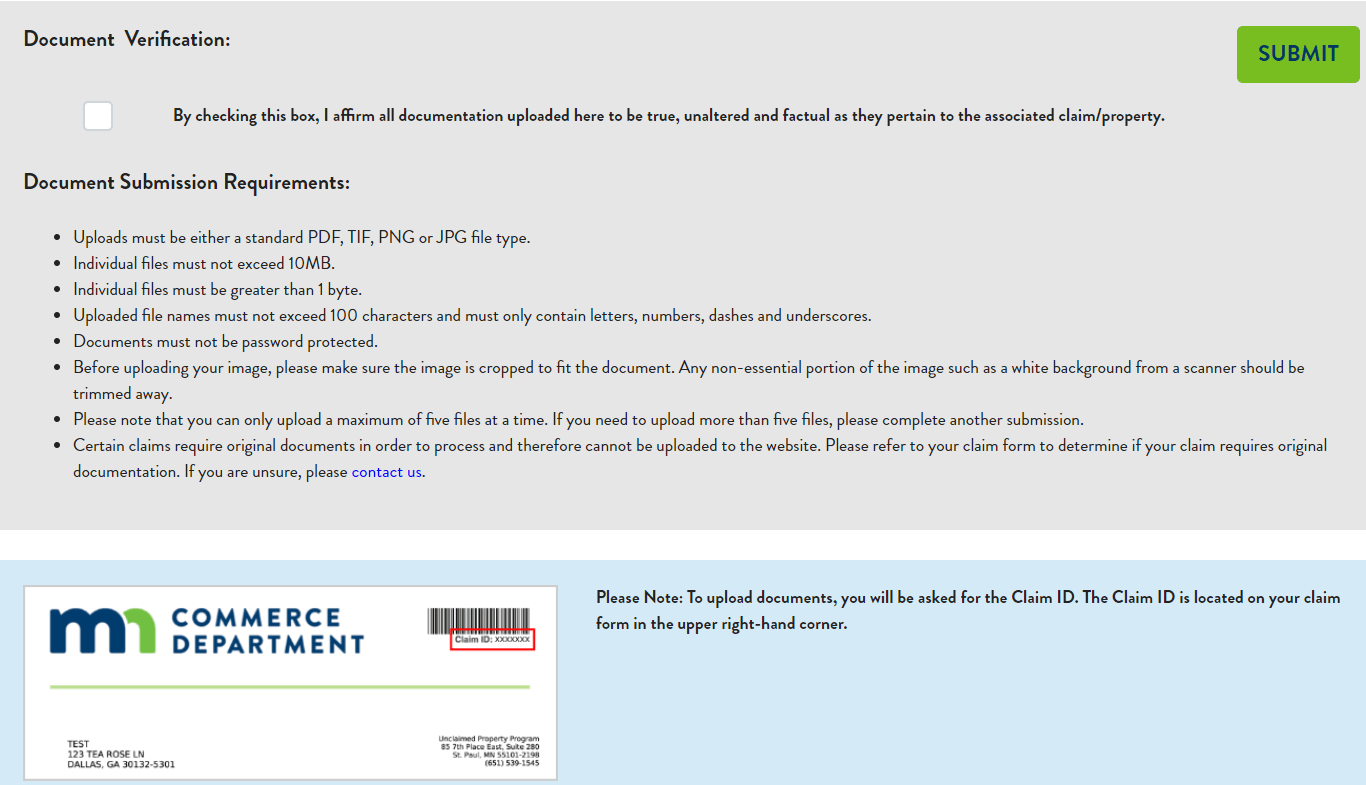The webpage displayed is dedicated to document verification and is divided into two main sections. The upper section, taking up about two-thirds of the screen, has a light grayish-purple background. In the upper left-hand corner, the title "Document Verification" appears in black text. 

Below this title, there is a white checkbox accompanied by a statement to its right: "By checking this box, I affirm all documentation uploaded here to be true, unaltered, and factual as they pertain to the associated property/claim." 

Further down, the heading "Document Submission Requirements" outlines several criteria for document uploads, including:
- Files must be in standard PDF, TIF, PNG, or JPEG format.
- Individual file sizes must not exceed 10 megabytes.
- Individual files must be larger than one byte. 

These requirements are presented in bullet point form for clarity. 

In the upper right-hand corner, there is a green "Submit" button with black text.

In the lower section of the page, there is an indication of a document that has already been uploaded, identified as originating from the "M Commerce Department."